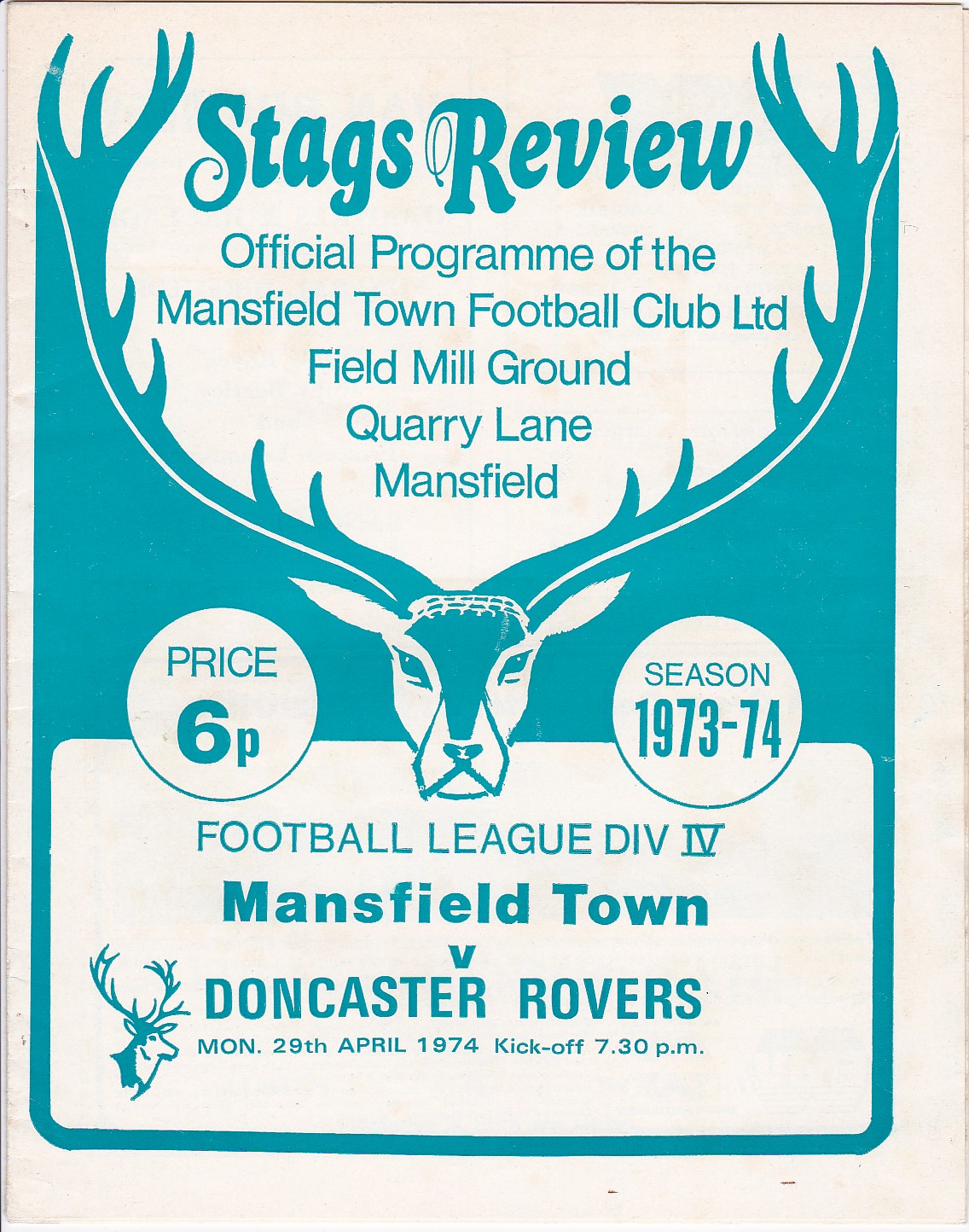The image is the cover of an old soccer program titled "Stags Review" in large bold letters at the top. It is an official program of the Mansfield Town Football Club Limited, for a match held at Field Mill Ground, Quarry Lane, Mansfield. Centered on the cover is a stylized, front-facing illustration of a deer head with large antlers extending towards the upper corners of the page. The text, which is in a greenish-blue color, is arranged between the antlers. To the left of the deer is the price, "6p," and to the right, the season, "1973-74." Below the deer, it reads, "Football League Division IV, Mansfield Town vs. Doncaster Rovers, Monday, 29th April 1974, kickoff 7.30pm." In the lower left corner, there is an additional small side view illustration of a deer head with its neck included. The design gives a vintage feel, capturing the essence of a soccer program from the era.